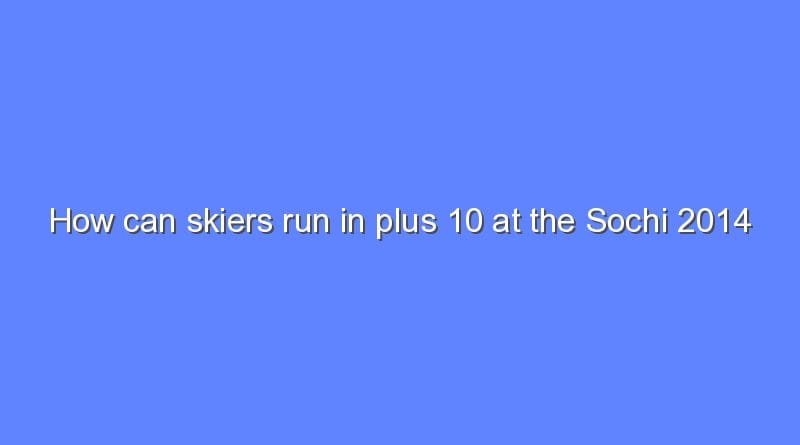The image features a periwinkle-colored square background with a slight purple hue. Centered perfectly within this bluish-purple backdrop is a line of white text styled in a Times New Roman font, complete with black shadowing for contrast. The text, which reads "How can skiers run in plus 10 at the Sochi 2014," is capitalized at the 'H' and 'S' and spans from the left edge to the right of the colored box, with ample spacing both above and below. This appears to be a slide from a PowerPoint presentation or similar visual medium, possibly serving as a prompt or a headline for further discussion.